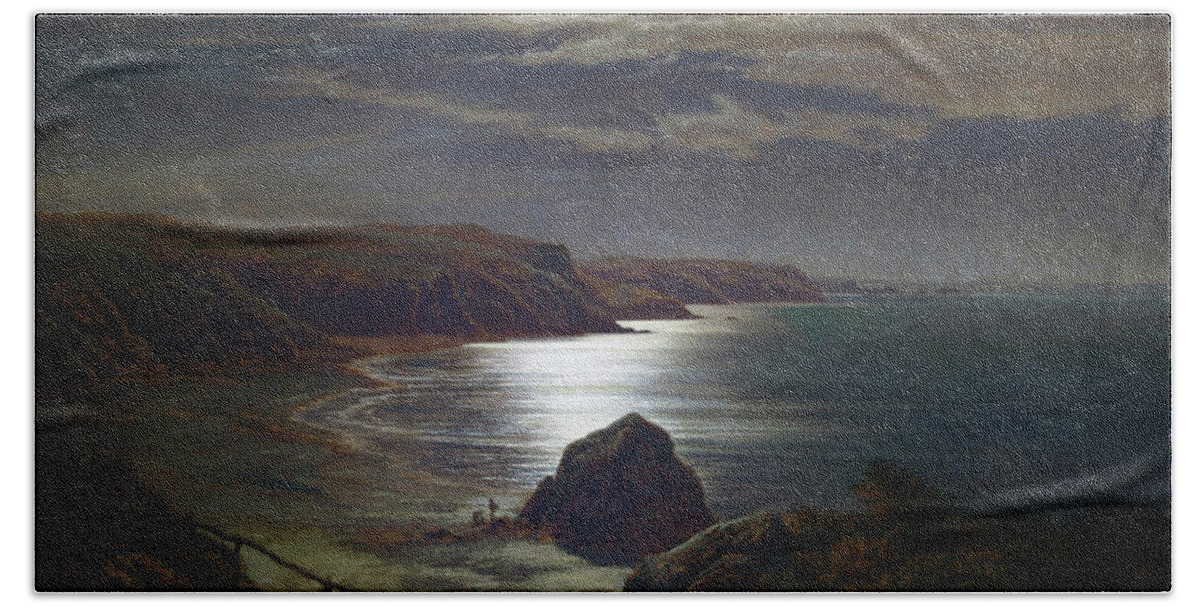The image is a very dark and grainy painting that depicts a nighttime coastal landscape. It features hilly terrain with flat-topped hills or natural rock faces alongside a large, still body of water. The water is calm, with only a few streaks of waves near the shoreline. A prominent boulder is situated at the center bottom of the painting, partially in the water. To the lower left, there's some vegetation, which could be either grass or a bush. The scene is enveloped in darkness, particularly around the rocks and grass, while the water reflects a mysterious, unidentifiable light source. The sky is overcast with clouds, adding to the enigmatic illumination of the water. The painting style appears to consist of textured dots rather than brush strokes. Despite the darkness, the moonlight brightens the ocean and the areas where the tide meets the shore. On the left side of the painting, brown cliffs can be observed, whereas the right side opens up to the vast expanse of the ocean. In the foreground near the boulder, there appear to be a couple of tiny figures, adding an intriguing element to the scene.